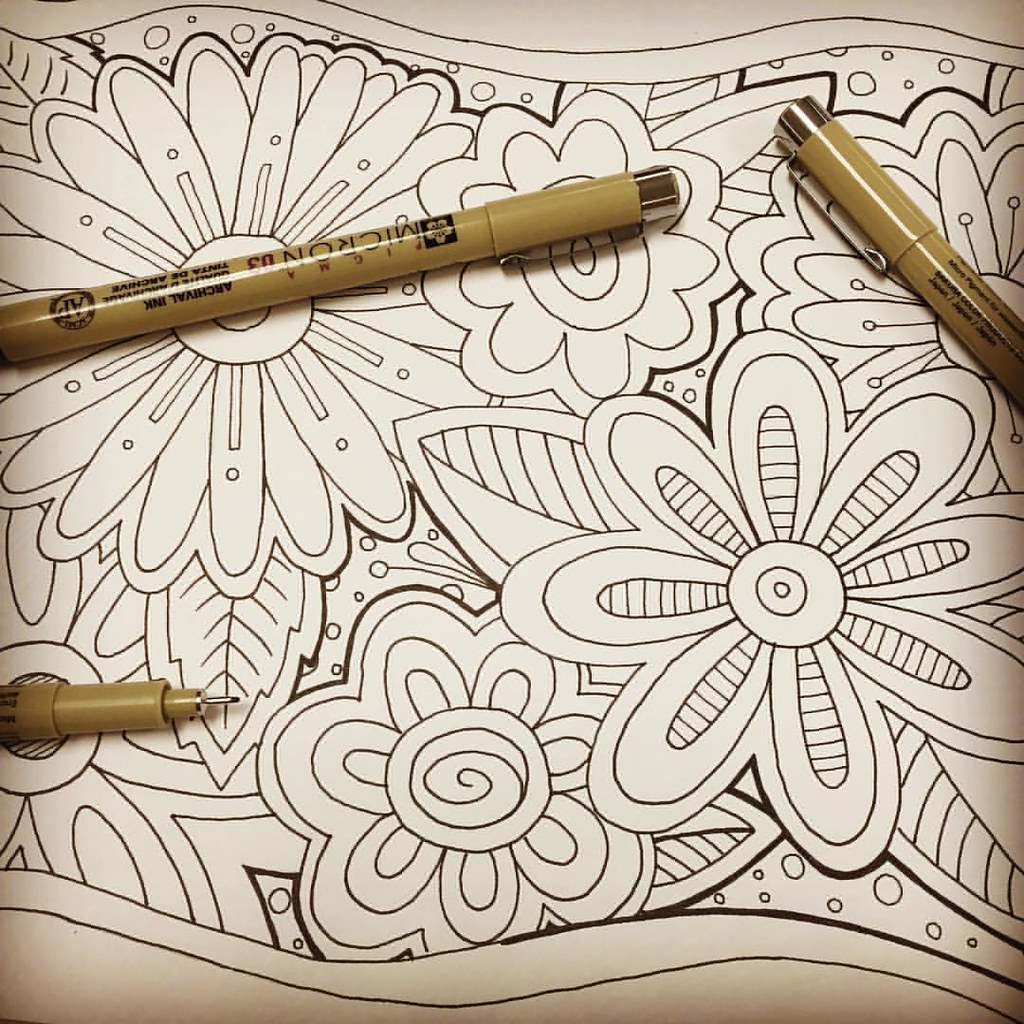The image features a detailed black-and-white floral design on an off-white or parchment-like background, typical of a coloring book page. The design includes six flowers, four of which are fully visible while two are partially cut off at the edges, all enclosed within a wavy, ribbon-like border. The flowers vary in shape, each with unique patterns within their petals, and are surrounded by simple greenery. On top of the image are three artist's pens, all in a light tannish color with reflective properties that make the writing hard to discern except for the labels "Picma Micron 03" and "archival ink." One pen has its lid off, laying near the bottom left, while the other two have their lids on positioned near the top. The overall scene suggests a tranquil, unfinished coloring activity awaiting a burst of colors.